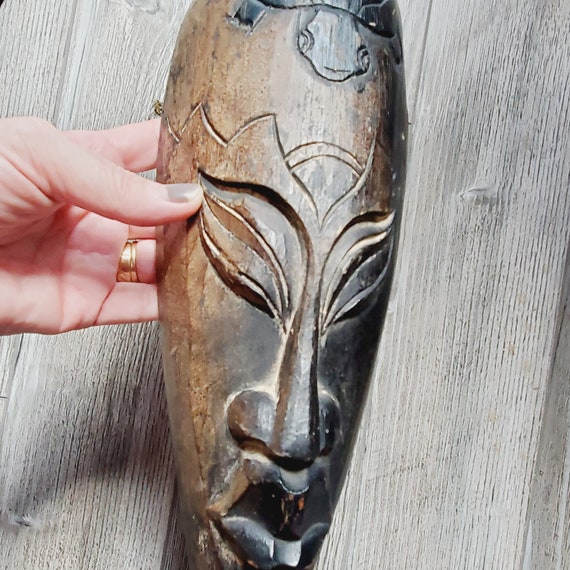The photograph showcases the left hand of an individual, adorned with a gold ring on the ring finger, holding an intricately carved, narrow wooden mask. The hand is palm side up, with the thumb securing the top part of the mask, while the other four fingers support it from beneath. The mask, characterized by its African style, is primarily brown and features a dark brown emblem on the forehead. Carved details form elongated, upward-angled eyes, a prominent yet flattened nose, and an open mouth with curved lips situated directly below the nose and at the base of the mask. The background consists of a surface and backdrops made of gray wooden planks, providing a rustic contrast to the rich brown tones of the mask. The oblong, oval-shaped mask is centered vertically within the square frame of the photograph.